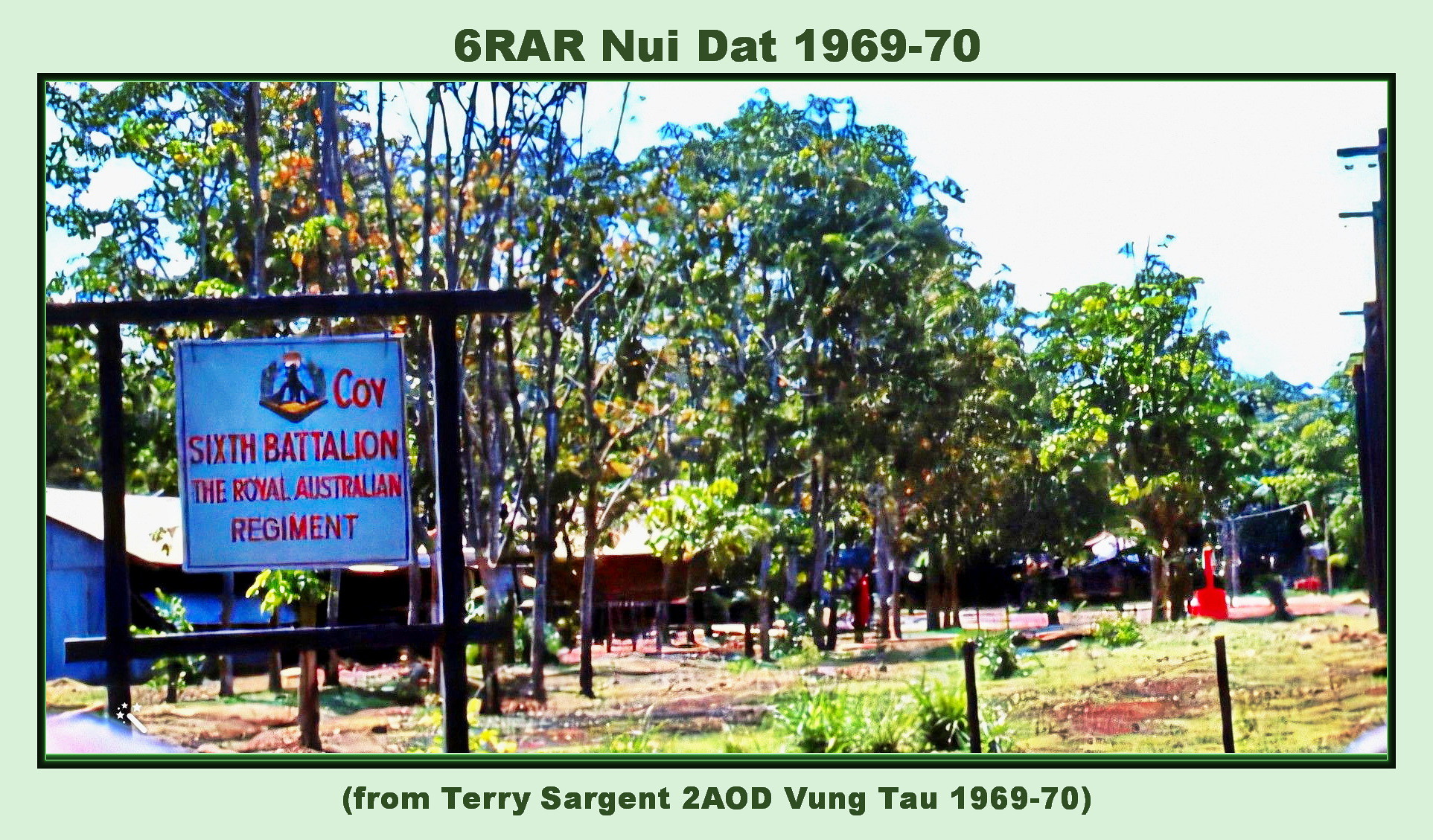The rectangular image with mint green borders presents a photograph captioned "6 RAR Nui Dat 1969-70" at the top and "From Terry Sergeant to AOD Vung Tau 1969-70" at the bottom. The bright, sunny scene showcases a base in Vietnam, featuring a grassy field and scattered trees. A prominent black wooden sign on the left, bearing the white and red inscription "Khoi 6th Battalion, the Royal Australian Regiment," stands out. Behind the sign, several small barracks can be seen, their roofs partially visible. The sky is bright blue, indicating clear weather, and the image is framed in widescreen dimensions, reminiscent of a high-definition TV.